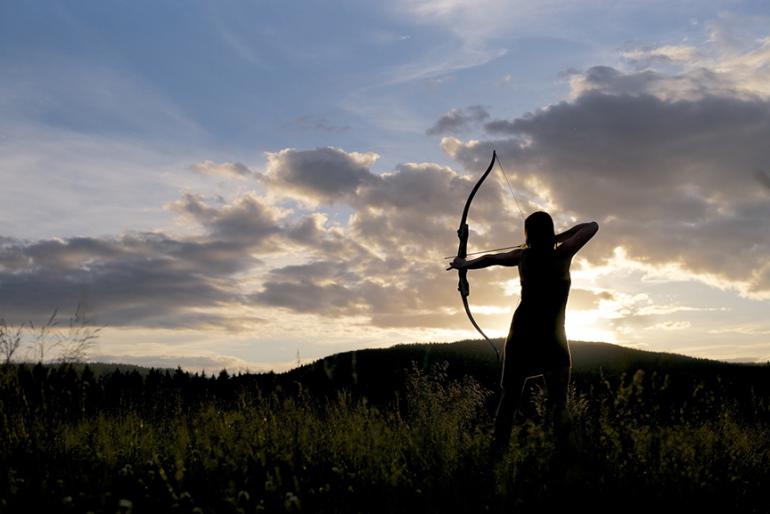At sunset in a field of tall grass, a silhouetted woman archer is captured in preparation to shoot an arrow. Her elongated right arm and arched elbow draw back a large compound bow, while her left hand extends the bow in front of her. The setting sun behind low hills casts the foreground in darkness, effectively masking the details of her figure, though you can discern her long brown hair and contours as she wears what appears to be a dress. The sky above is predominantly blue, densely populated with gray clouds, enhancing the dramatic atmosphere of the scene. The background features a hilly terrain, adding depth to this serene outdoor moment.